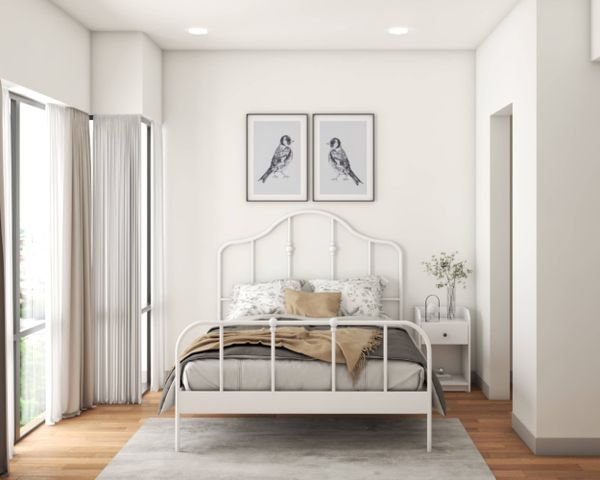The bedroom features white walls and a light-colored wooden floor, creating an airy and clean aesthetic. Dominating the room, a four-poster bed boasts a combination of bedding: a gray cover, a tan fringed blanket, and a tan pillow that matches the blanket. Behind this central pillow, two white pillows further accent the bed. A pair of black-and-white bird illustrations, showing birds facing each other, hangs above the headboard. To the right of the bed, a white nightstand with a black knob holds a vase with white and dried flowers. The bedroom's lighting includes two recessed, white ceiling lights. To the left of the bed, sliding glass doors with white vertical blinds (currently open) and surrounding curtains provide access to what appears to be a grassy yard. A gray, silverish area rug rests beneath the bed, adding texture to the room's predominantly white and wood-toned decor. Lastly, to the right of the bed, there is a doorway likely leading to the bathroom.